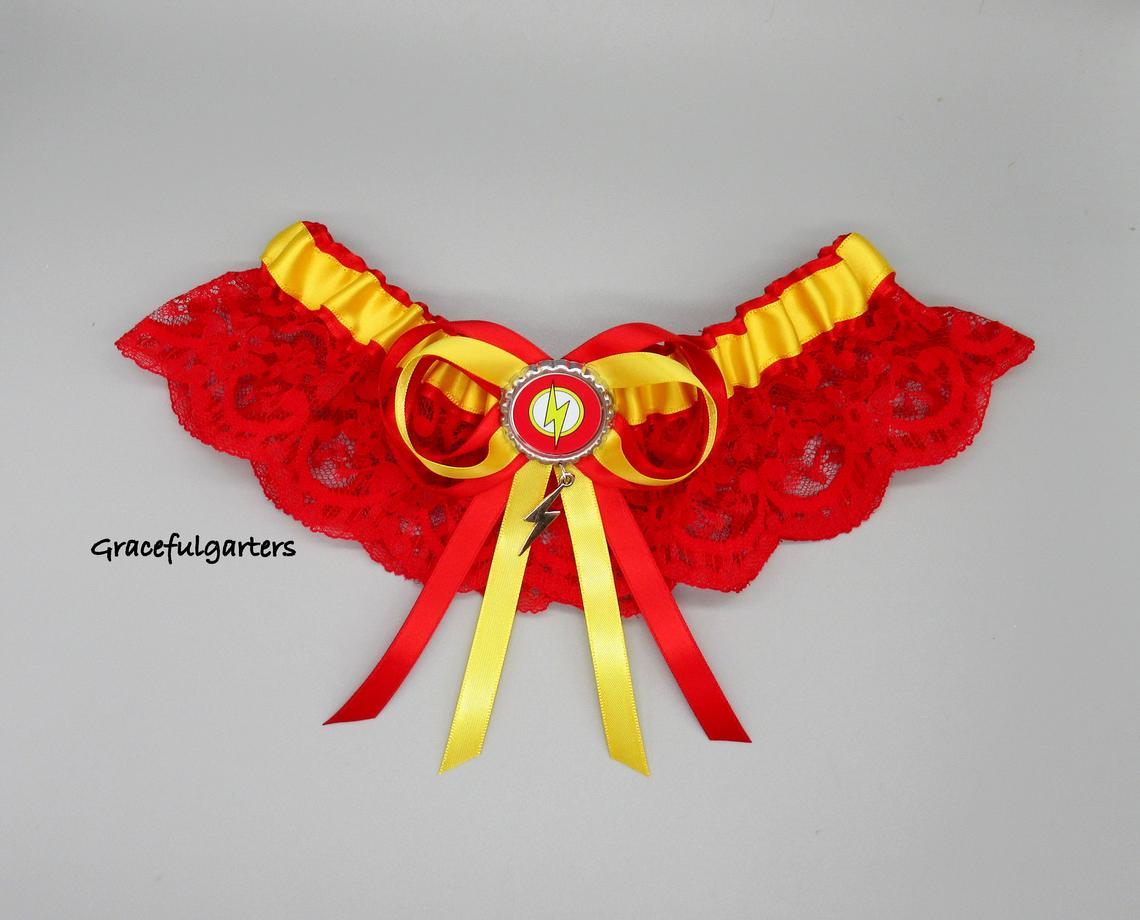This image features a detailed, decorative garter belt likely intended for women. The garter is crafted from lace with a rich red color, adorned with an intricate border that is a gold or yellowish hue. At the center of this elegant accessory is a striking bow made from the same gold-colored lace. Prominently displayed in the middle of the bow is an ornate pendant. This pendant has a silver edging and showcases a series of nested circles: a red outer circle, a yellow middle circle, and a white inner circle. At the very center of the white circle is a vivid yellow lightning bolt. Additionally, the garter has four extending ribbons: two red ones that slant downward and two yellow ones that fall more vertically. The image also includes text to the left that reads "Graceful Garters," likely indicating the brand name. The garter is arranged on a gray surface, highlighting its vibrant colors and elaborate design.